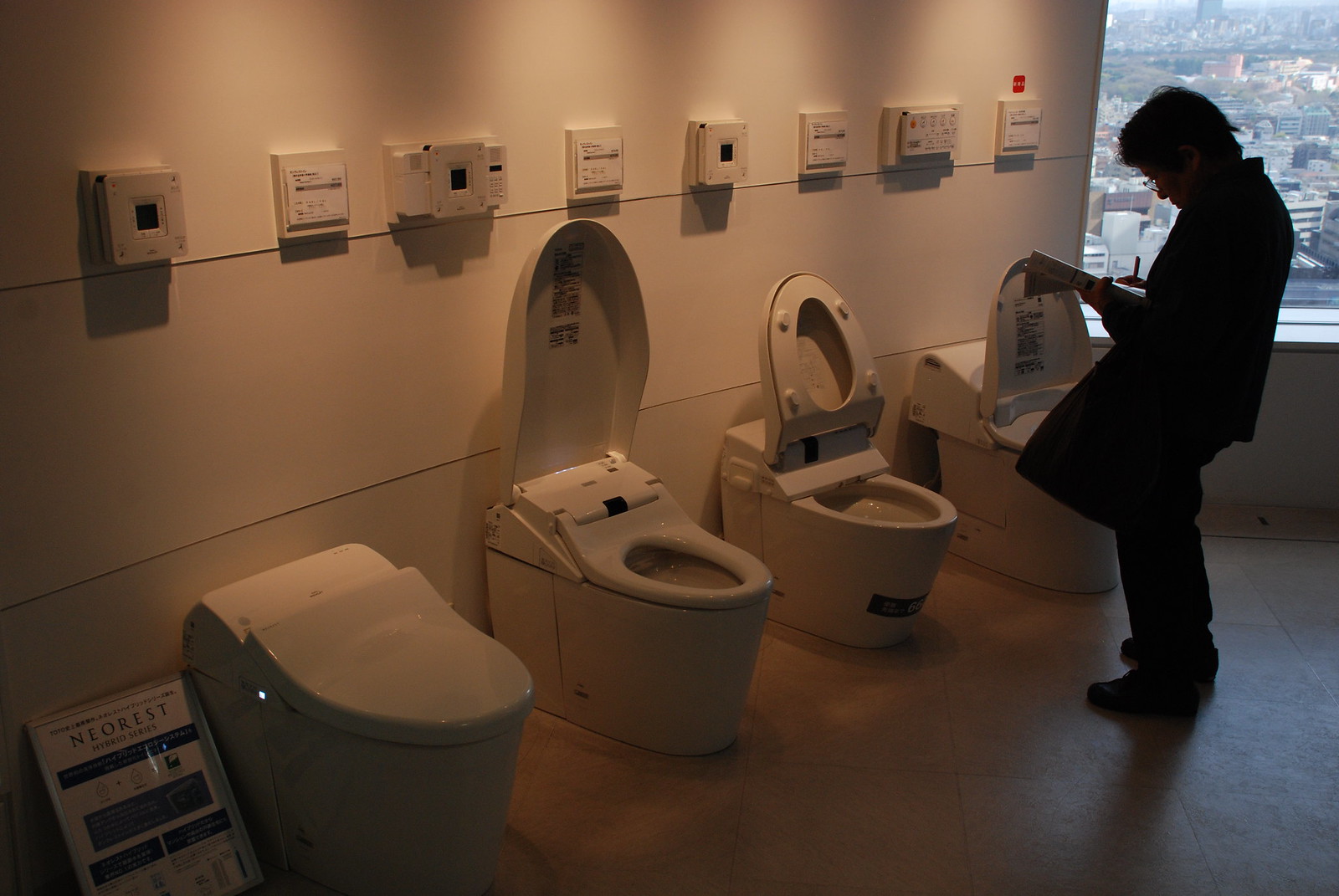The image depicts a high-floor showroom with a view of the cityscape through large windows, featuring four large, bulky, self-contained toilets arranged in a row against the wall, each with very wide bases and sizeable lids. The first toilet from the left has its lid closed, the second one has its lid open, the third has both its lid and seat open, and the fourth toilet has its lid closed. Above each toilet, there are electronic devices mounted on the wall with screens and attached sheets of paper providing information. A man, dressed in all black and wearing glasses, stands in front of the second toilet from the right, slightly bending as he reads or takes notes from a piece of paper in his hand. The room has a linoleum floor, enhancing its showroom-like appearance.